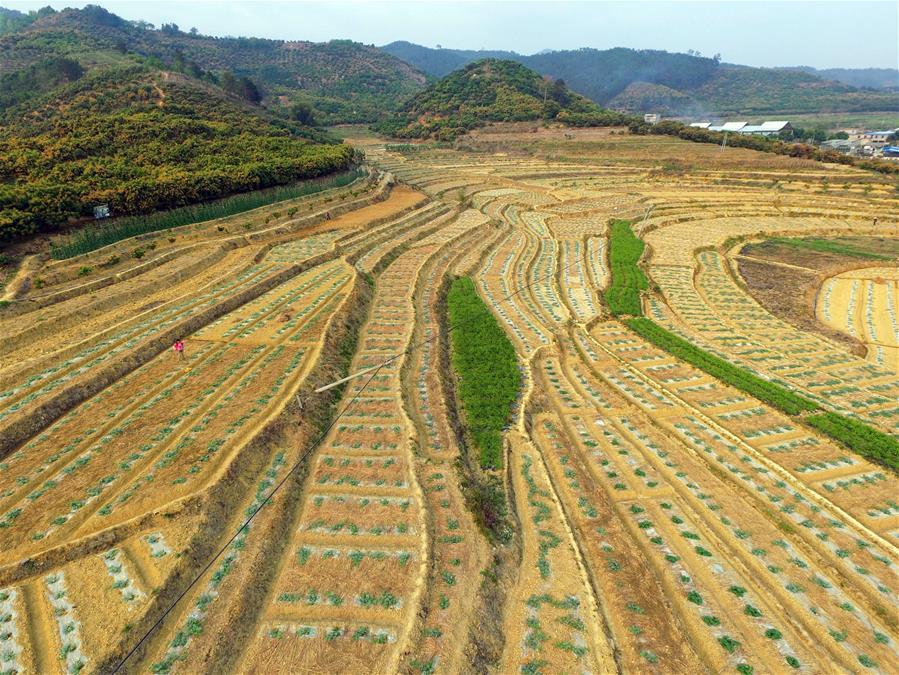The image depicts a vast, tiered farming landscape that appears to be reminiscent of agricultural fields often seen in Asia. At the center-left of the image, a person dressed in a bright pink outfit stands out, possibly engaged in some fieldwork or photography. The terrain is filled with rows of green plants arranged in various orientations—some vertical, others horizontal—on narrow tiers that slope upward from right to left. The ground between these tiers is predominantly brown, indicative of dirt or perhaps recently planted crops.

In the background, there are elevated mountains and hills filled with lush greenery, creating a stark contrast to the more sparsely vegetated field below. The scene suggests a warm climate, characteristic of spring or summer, and the vibrant landscape is free from buildings except for a few with white roofs visible at the top right corner of the image. This picturesque, colorful setting, with its layered cultivation and distant verdant hills, paints a vivid picture of agricultural life amid natural beauty.